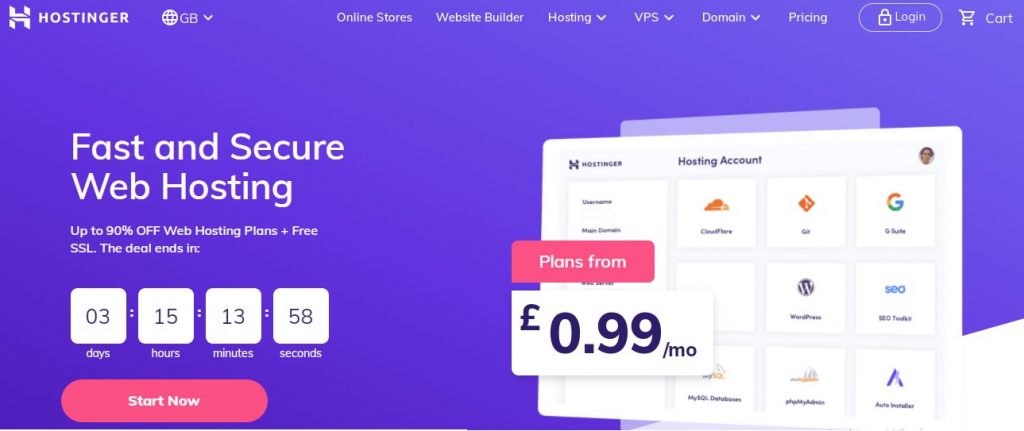**Screenshot Description: Hostinger Web Hosting Offer Page**

The screenshot captures Hostinger's web hosting offer page. The image has a dark blue background in the top left corner. Prominently displayed in this area is the big, bold letter "H" followed by "HOSTINGER" in all capital, bold letters.

To the right, there's a circle with vertical white lines inside, next to which is "GBM" in white letters. About an inch to the left, the header navigation features various menu items including "Online Stores," "Website Builder," "Hosting" with a drop-down arrow, "VPS" with a drop-down arrow, "Domain" with a drop-down arrow, and "Pricing." Further to the right, there's a blue tab with a white border featuring a white lock icon and the text "Log In." To the left of this tab, there is a white shopping cart icon with the word "Cart."

If you scroll down about two inches, a white pop-up square appears on the left side, showcasing "Hostinger" in black text at the center. The right side mentions "Hosting Account" with a profile picture below it. Below this are four rows of icons, each accompanied by descriptive text.

In the center-left of the image, a pink tab with white text reads "Plans from." Below this is a larger white square with "€0.99/MO" in bold on the left side. Directly underneath the "Hostinger" logo, and about halfway down, large bold white text reads "Fast and Secure." Below this in smaller white text, it states "Up to 90% off web hosting plus free SSL." This is followed by "The deal ends in," followed by four squares indicating time left for the deal: "Days," "Hours," "Minutes," and "Seconds." Currently, these boxes display "03," "15," "13," and "58" respectively. Below these countdown boxes is a red tab with white text that says "Start Now."